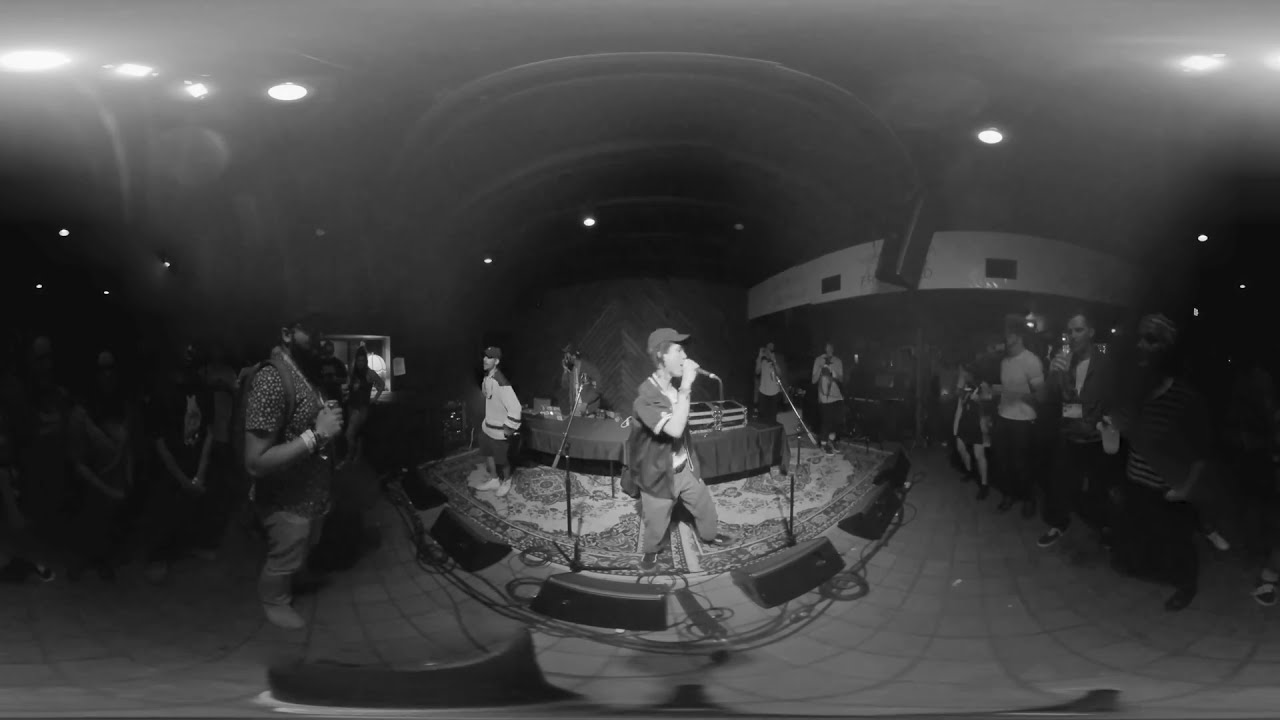This black-and-white panoramic photo captures a dynamic concert scene. At the center, two performers dominate the frame, one actively singing or rapping into a microphone while the other holds a mic in his left hand and gazes at the crowd. The singer, wearing a black shirt and cap, stands on a patterned mat, illuminated by spotlights from above. To his left, the second performer, also wearing a cap but in a lighter shirt, stands on the same level as the audience, who are separated by a modest space yet fully attentive, drinks in hand. To the right of the performers, there's a DJ or another participant wearing headphones and potentially holding a notebook. The stage is surrounded by speakers, and the audience frames the scene on both sides, amplifying the energy of the moment. The ceiling's darkness contrasts starkly with the bright spotlights, which cast a sharp focus on the central figures while leaving the spectators in relative obscurity. Adding to the milieu, an observer with a camera is also capturing the event.